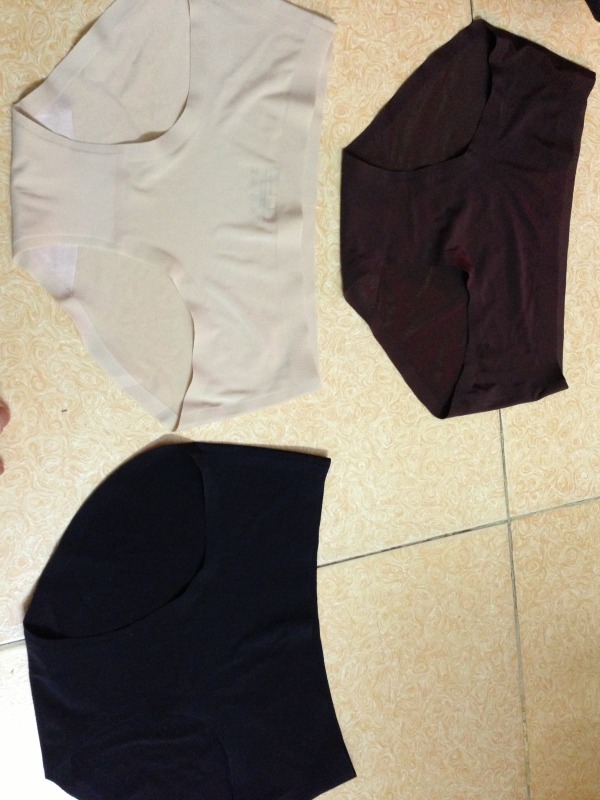In this color photograph, taken in portrait orientation from a standing position, a tiled floor with large, golden-beige tiles serves as the backdrop. The tiles create a grid-like pattern and host three pairs of women's underwear, all plain and no-show seamless, lying flat and prominently displayed. At the top of the image are two pairs of briefs: one on the left, which is an off-white color, wrinkled and showing signs of wear; and another on the right, a very dark shade close to burgundy, almost black. Below them in the lower left corner of the photo is a third pair, which is entirely black. Each pair is positioned with the crotches pointed left. A small, barely visible reddish-orange object is partially seen on the left side of the frame, adding a subtle yet intriguing detail to the composition.